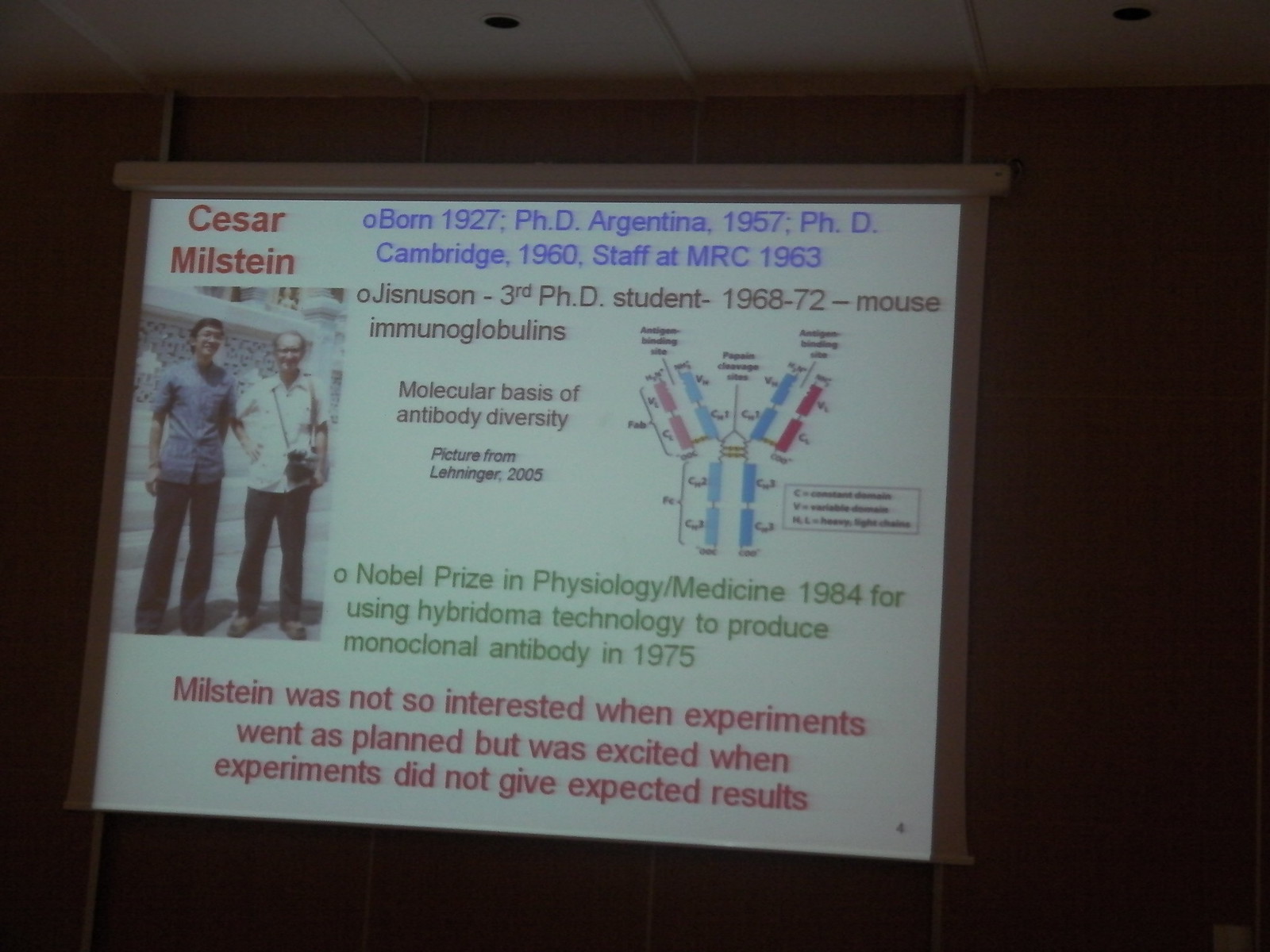This is a wide rectangular image of a projector screen displaying a PowerPoint slide. The photograph captures part of the off-white tile ceiling at the top, while the rest of the image is dark. The screen is positioned slightly left of center, held by a white metal rod at the top. The PowerPoint slide, set against a white background, prominently features a tall, rectangular photograph of two men standing side by side on the left. Above the photograph, "Cesar Milstein" is written in red font. To the right of the image, blue text details Milstein's credentials and career milestones: "Born 1927, Ph.D. Argentina, 1957, Ph.D. Cambridge, 1960, Staff at MRC, 1963." Below this, additional black text reads: "Just Newsom, third PhD student 1968 to 72, Mouse Immunoglobulins." The slide also includes a diagram illustrating the molecular basis of antibody diversity. In green text, it notes: "Nobel Prize in Physiology/Medicine 1984 for using hybridoma technology to produce monoclonal antibodies in 1975." At the bottom of the slide, red text states Milstein’s unique enthusiasm for unexpected experimental results: "Milstein was not interested when experiments went as planned but was excited when experiments did not give expected results."